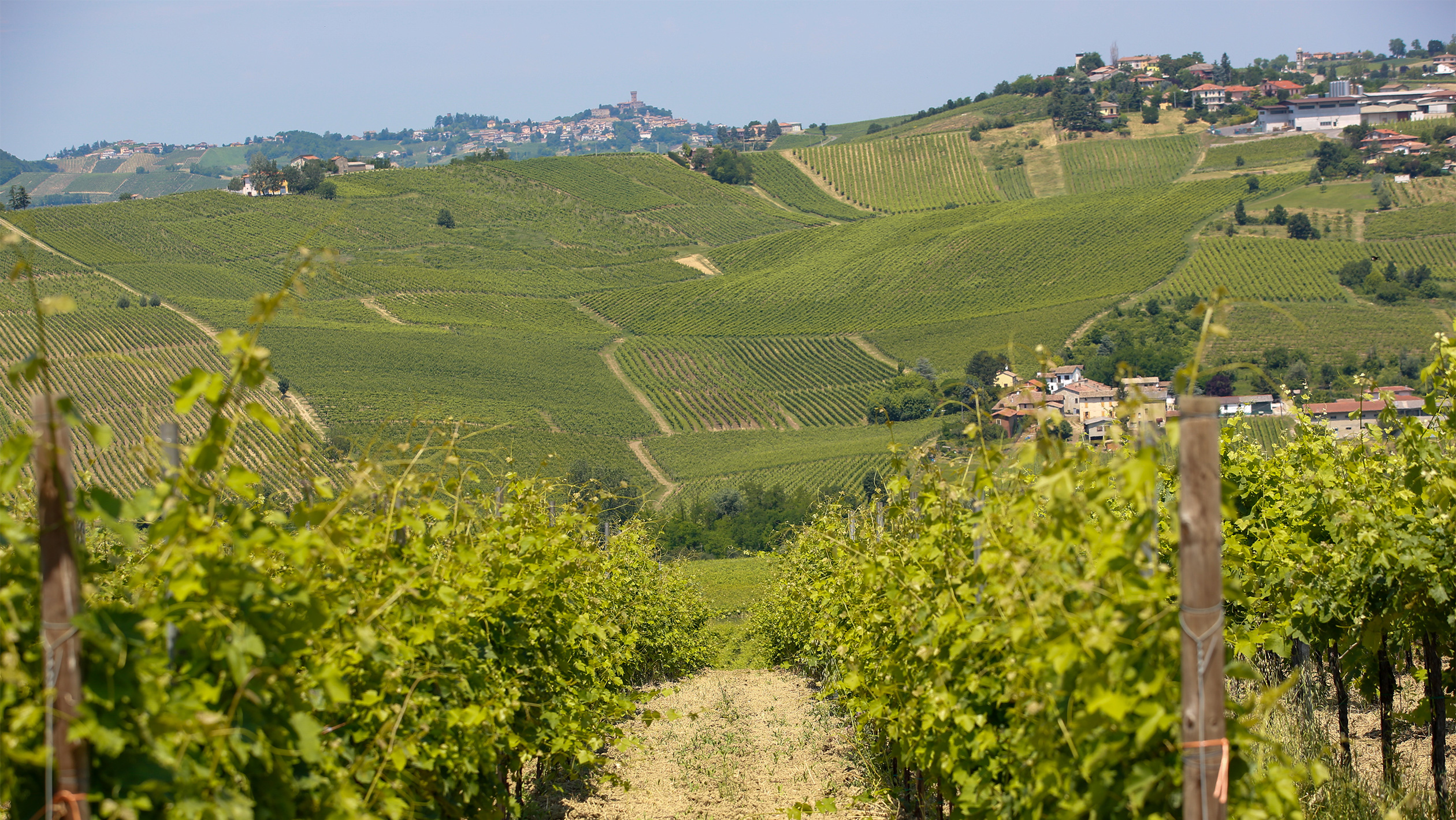The landscape photo captures a vibrant and orderly vineyard stretching from the foreground to the background. Central to the image is a dirt road flanked by carefully maintained grape vines. The greenery is lush, with an array of green trees scattered throughout the scene. The fields are well-tended, showing vertical lines indicative of crop cultivation. On the middle right, a quaint village with a cluster of houses nestles amidst the hills, while the far background reveals a larger city complete with a prominent building perched atop a hill. The blue sky arches over the entire scene, enhancing the vivid green of the vineyard and trees, and the dry, light brown dirt road running through the center. The left side of the image also contains some light-colored buildings interspersed with more green vegetation, adding to the pastoral charm of the landscape.